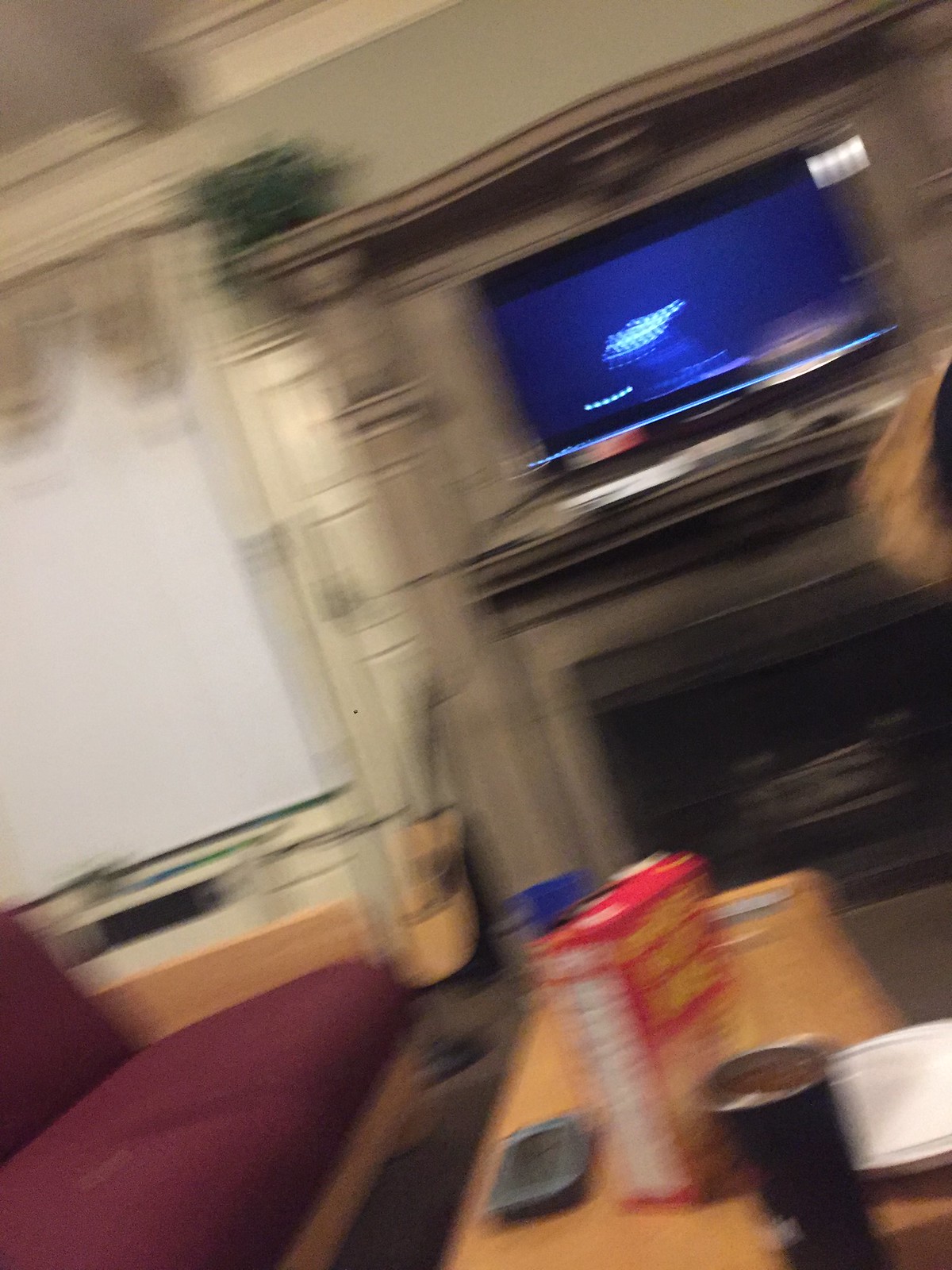The image depicts a detailed view of a living room with a distinct light green to gray color on the back wall. Central to the room is a gray fireplace with a large mantel above it. Positioned on the mantel, directly above the fireplace, is a television displaying a blue screen with white lights. Adjacent to the fireplace on the left is a tan guitar with a black handle, leaning against the wall. Directly in front of the fireplace stands a light brown wooden coffee table, which holds a variety of items: a red box of cereal with yellow writing, a dish or plate, a black cup, and a cell phone. To the left of the setup, there's a burgundy sofa that matches the wood and fabric blend of the room's decor. Behind the coffee table, to the left, there are window coverings, including white blinds and a white or light gray valance. A barely visible person, with blurred hair, is passing through the right side of the photograph, adding a dynamic element to the otherwise static scene.